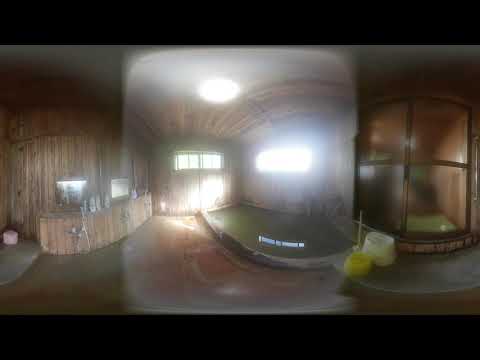The image depicts the dimly lit interior of what appears to be a rustic, old building, evocative of a time-period setting one might see in a video game. The walls and ceiling are adorned with weathered, rustic wood paneling, giving the space a warm, log cabin or spa-like atmosphere. On the left side, there is a counter area with bath products, reminiscent of a bar or reception area. Below the counter are a yellow and white bucket and an upright mop, suggesting ongoing maintenance or cleaning. Moving toward the right, a recessed ceiling light illuminates the center of the room, highlighting a small, four-paned window that allows light to filter in. Further along the right wall, there is a shallow, in-ground tub, which could easily be mistaken for a pond, adding to the room’s log cabin sauna vibe. Adjacent to this tub, glass doors may lead to a shower or sauna area. Surrounding these doors are baskets or containers on a small rug. Overall, the room exudes a spacious, rustic charm, with multiple windows allowing soft natural light to seep through, enhancing the serene ambiance.